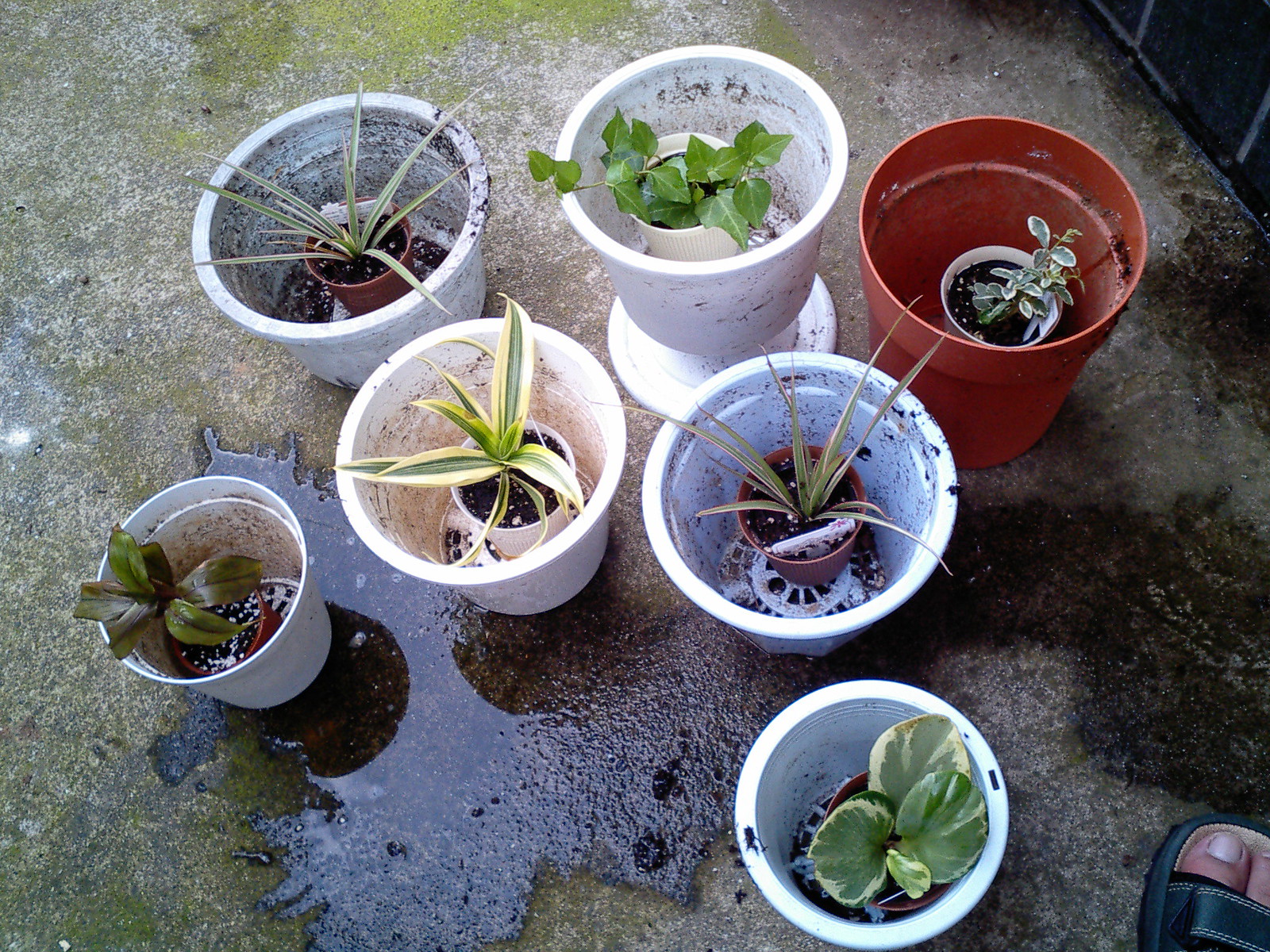This is a detailed aerial photograph taken outdoors, capturing seven planters arranged on a concrete surface, which is sprinkled with green moss and small puddles of water. The photo includes a person's big toe in a black sandal at the lower right corner. Each planters features a distinctive plant within a smaller pot nestled inside a larger pot. Most of the larger pots are white plastic, except for one terracotta-colored pot.

At the top of the image, there is a row of three planters: a white planter holding a small spider plant, another white planter containing an ivy plant with multiple green leaves, and a terracotta-colored planter housing a plant with green leaves edged in white. Below this row are two more white planters; the one on the left also contains a spider plant, while the one on the right's contents are unspecified. Further down and separate from the rest, lie two smaller white planters; the left one holds a plant with green leaves tinged with reddish coloring, and the right one contains a plant with round green leaves marked with white. The plants are vibrant and healthy amidst some loose soil and minor water splashes, suggesting they are either ready for purchase or recent care.